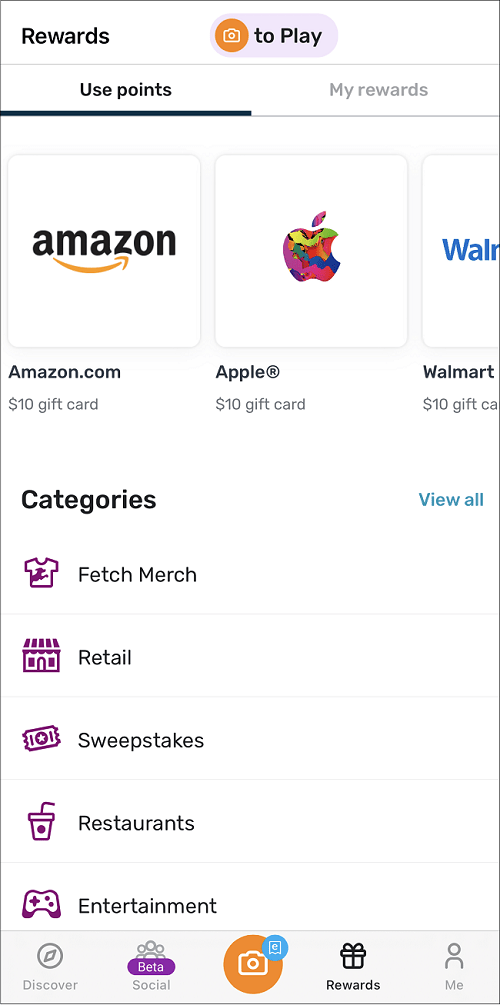The image showcases a mobile device screen displaying a page from the Fetch app.

At the top, the page is titled "Rewards" with an orange circular camera icon labeled "To Play" beside it. Below that are two tab sections: "Use Points" (highlighted in black with an underline, signifying it's selected) and the grayed-out "My Rewards."

The "Use Points" tab reveals a section displaying various gift card options:
1. Amazon - a square featuring the Amazon logo, offering a $10 Amazon.com gift card.
2. Apple - a square with the Apple logo, offering a $10 Apple gift card.
3. Walmart - a partially visible square showing "WAL" in blue text, indicating a $10 Walmart gift card.

Beneath the gift card options, a "Categories" section is listed in black text, accompanied by a blue “View All” link. The categories include:
- "Fetch Merch" with a purple shirt icon.
- "Retail" marked by a purple building icon.
- "Sweepstakes" indicated by a purple ticket outline.
- "Restaurants" represented by a purple cup outline.
- "Entertainment" with a purple game controller outline.

At the bottom of the screen, a navigation bar displays five icons:
- "Discover"
- "Social" (with a "Beta" label)
- "Camera"
- "Rewards"
- "Me"

This detailed layout provides a clear view of the various sections and options available on the Fetch app's rewards page.